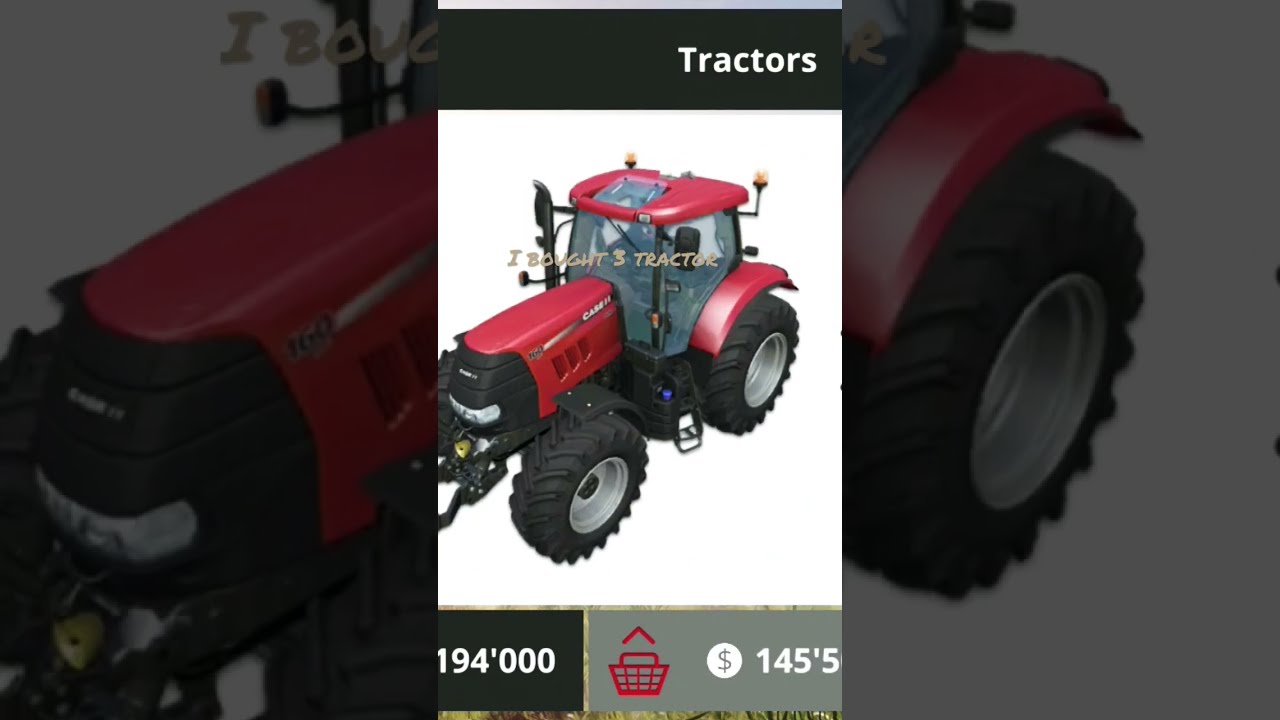The image is a vertical cell phone screenshot of an advertisement for a red tractor, displayed against a pure white background. The image is flanked by heavily tinted, zoomed-in sections of the same tractor, with the left side focusing on the front grill and the right side on the back tire. At the top of the image, a black rectangular border contains white text on the right that reads "TRACTORS" in all caps. The central tractor, viewed from a front corner at a slight elevation, features large black-trimmed tires with gray rims, red fenders, and partially open sides. On the front of the tractor, light brown handwriting text states, "I bought three tractor." At the bottom of the screenshot, there's a black rectangle displaying the number "194,000" and a gray rectangle next to it with a red shopping basket icon and the text "$145.5" alongside a dollar sign. The image leaves some ambiguity about whether the tractor is life-sized or a miniature model.